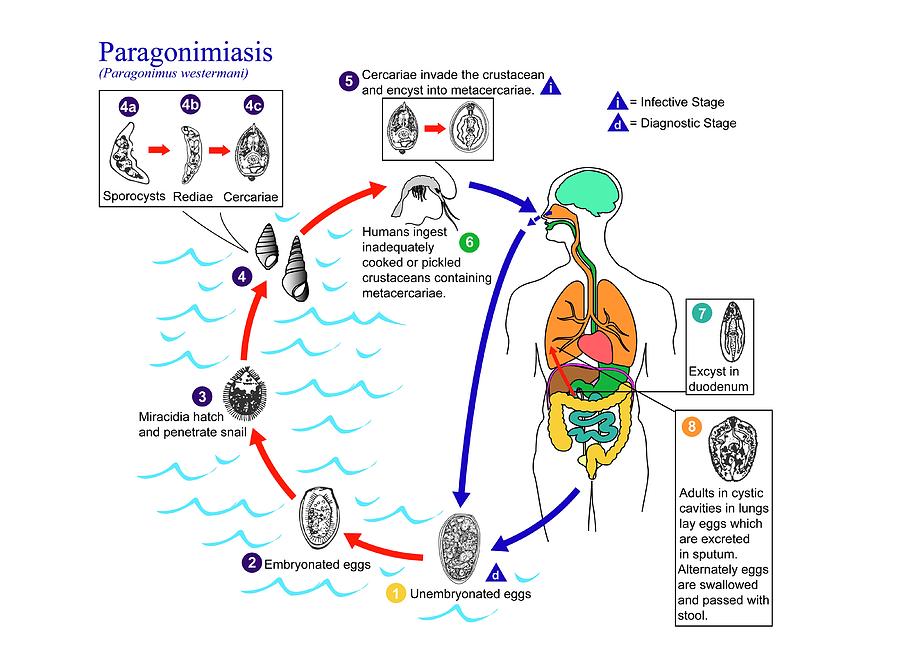This detailed diagram illustrates the transmission cycle of a disease that humans can contract from crustaceans. It features a transparent outline of the human body, revealing the internally affected organs in vivid colors. Each organ affected by the disease is clearly labeled. The life cycle of the disease is meticulously charted, starting with eggs that infect a snail. The infected snail is then consumed by a shrimp, which subsequently gets ingested by a human, completing the cycle. Each stage, from the eggs to the snails, shrimps, and finally to the human, is marked and described with labels, providing a clear and comprehensive understanding of the disease's progression and transmission.